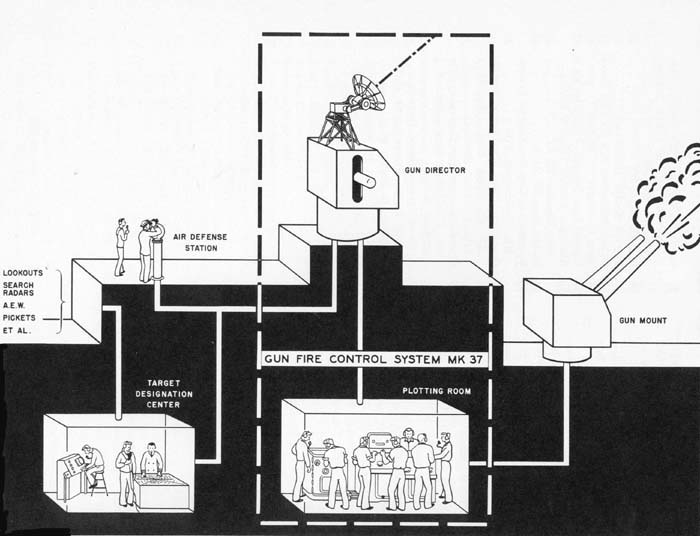The image is a detailed, black and white, computer-generated cutaway drawing of a large structure, likely a ship, showcasing a gunfire control system MK 37. The central focus is a labeled room indicating "Gunfire Control System," populated by approximately seven men operating various dials and machinery. Above this, the section is labeled "Gun Director," and to the right, a "Gun Mount" is depicted, showing double cannons firing with lines indicating smoke. To the left, an area marked "Air Defense Station" features two men, possibly using binoculars. Below this, the "Target Designation Center" displays three individuals engaged in plotting or dialing in target coordinates. Additional sections, including "Lookouts, Search Radars, AEW, Pickets, et al.," are labeled throughout the landscape, emphasizing the multifaceted nature of this complex weapon system. This illustrative cutaway provides an in-depth view of the intricate operations and personnel involved in this gunfire control system.